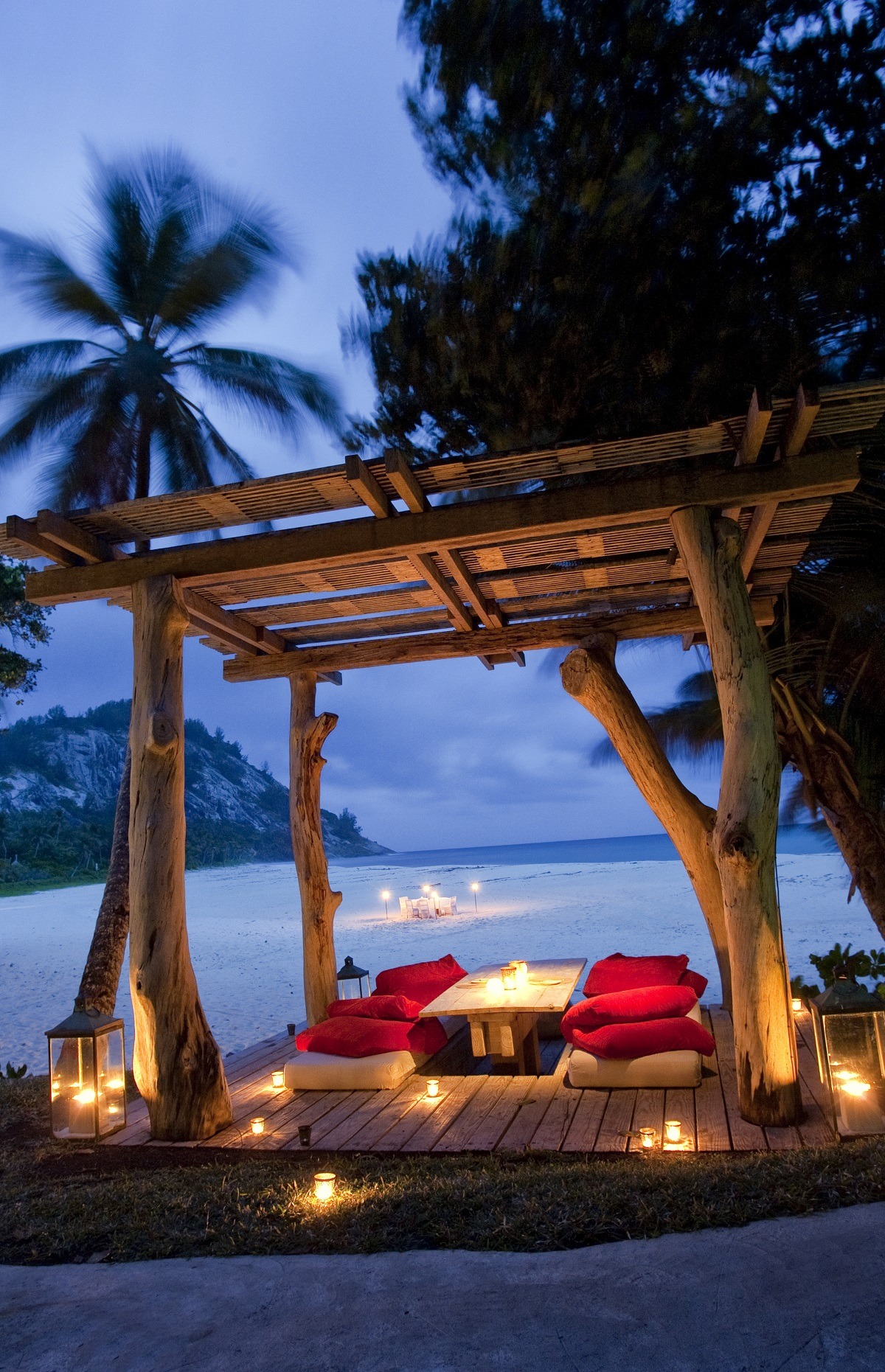The image is a vertically aligned digital photograph taken outdoors near a body of blue water in the early evening. The scene captures a charming, candlelit seated area set on a sandy beach with a stone pathway. Two small white beds with red pillows are positioned on either side of a wooden table adorned with three lit candles. Additional candles are scattered around the area, casting a warm, yellow glow. In the background, another candlelit setup suggests a campfire setting. To the left, a small cliff with green bushes or trees adds a natural touch. Towering palm trees frame the top of the picture against a still-lit evening sky. The colors in the image range from light blue and dark blue to white, gray, black, tan, and red, creating a serene and inviting atmosphere.